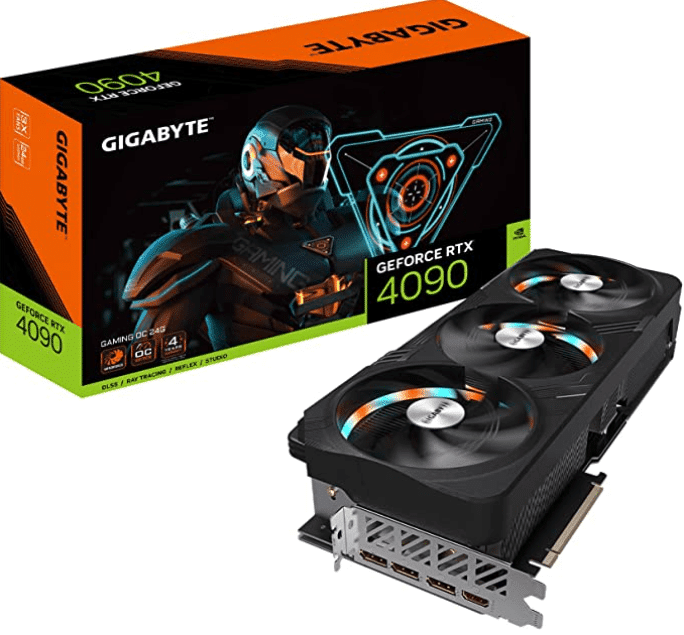This is a highly detailed promotional image for the Gigabyte GeForce RTX 4090, one of the top-tier graphics cards available on the market. The image features both the product itself and its packaging. On the left, the box is predominantly black with orange and green accents, along with some blue neon highlights. The front of the box prominently displays the Gigabyte logo at the top, "GIGABYTE" (spelled out), and the model name "GeForce RTX 4090" at the bottom right corner. Also present on the box is "Gaming OC 24G" and additional design specifications.

In the middle of the box, there's an illustration of a highly armored, futuristic soldier. This character, reminiscent of a figure from Halo, is depicted interacting with a blue and orange triangular hologram. The soldier has "Gaming" inscribed on its chest plate, adding a gaming-centric appeal.

To the right of the box is the actual graphics card, which is massive and appears to occupy around two PCIe slots. The card itself is black with a robust plastic encasement and a silver metal bracket on one side where the connectivity ports are situated. The card also features three large cooling fans with RGB lighting, creating a blur effect, appearing as if the blades are spinning, emitting white, blue, and orange light. Additionally, the card includes various display ports, including two DisplayPorts and two HDMI ports.

The overall scene is set against a white background, which emphasizes the product, making it suitable for an advertisement or an online retail listing.